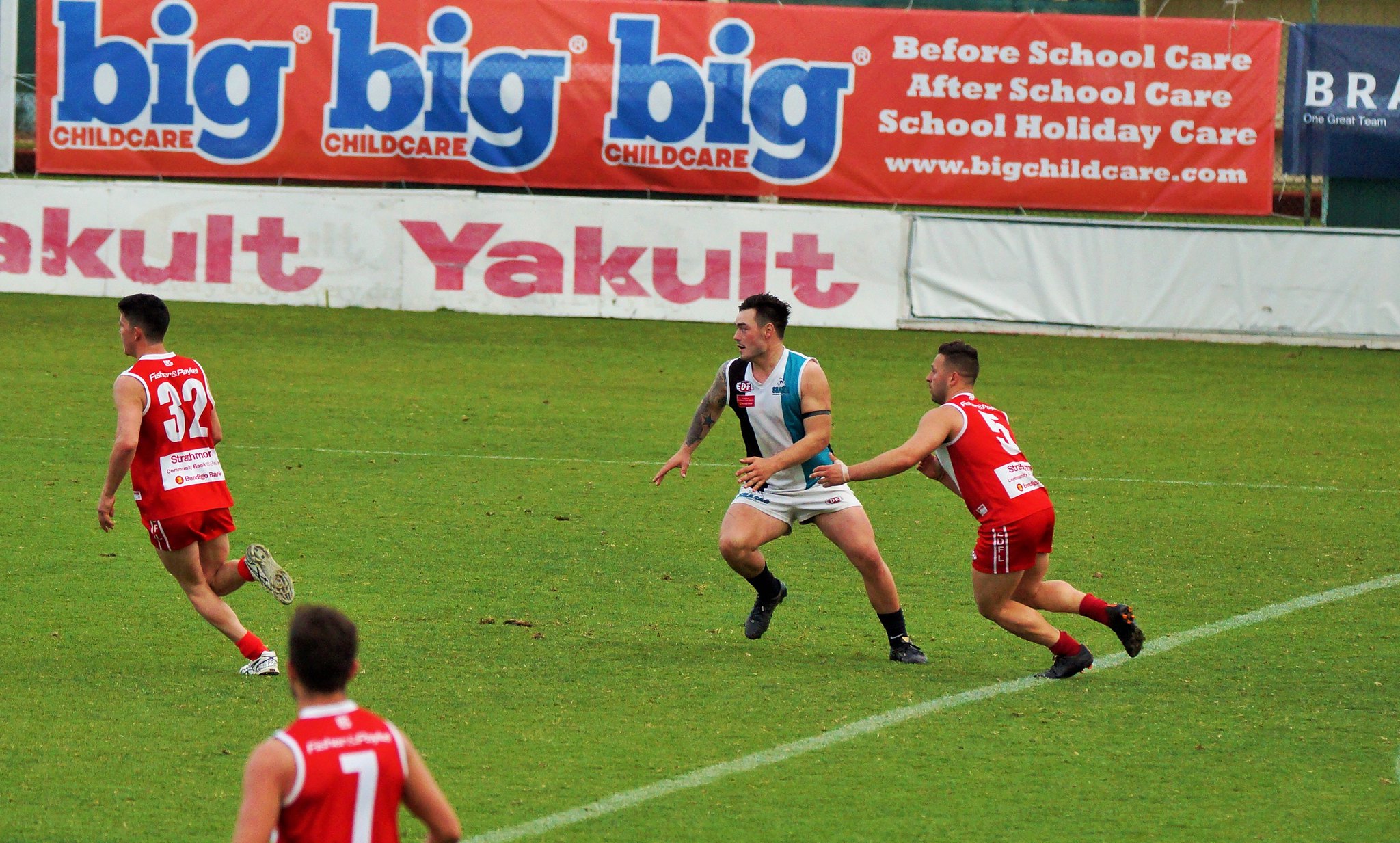In this dynamic action shot taken on a green soccer field, four men are captured in the midst of a game. Three players don red, sleeveless uniforms, while a fourth player stands out in a white and blue striped jersey with matching white shorts. Their intense focus is directed towards an unseen ball coming from the left side of the frame. The green field features a white stripe along its edge, further adding to the scene's vividness. In the background, advertisements cover a white wall; one prominently displays "Ya Cult" in bold red letters. Another large red banner reads "Big Child Care" in blue letters, followed by details in white about their services: "Before School Care, After School Care, School Holiday Care," along with a website URL. The players' attire—including sleeveless jerseys, short shorts, and tattoos—suggests they may be rugby players, though the context implies a soccer match. This descriptive snapshot captures the intensity and atmosphere of the game, set against a backdrop of vibrant advertisements.